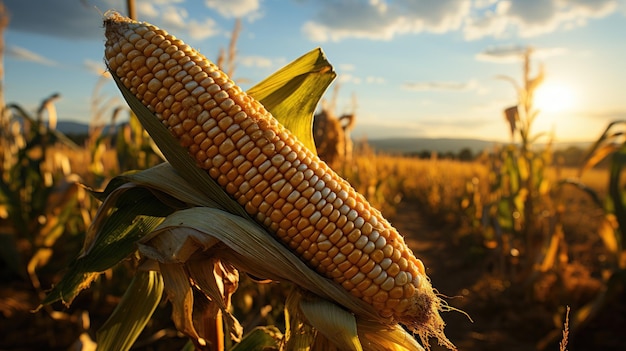This image depicts an ear of corn in striking detail, prominently set against a backdrop that fades into a blurred cornfield and mountains on the horizon. The corn, meticulously peeled to reveal each individual kernel, features a mixture of honey gold and lighter yellow shades suggestive of varied ripeness, akin to Indian corn with its hard kernels. The visual contrast between the sharply focused corn and the blurred surroundings adds depth to the scene. The husks, a pale greenish-gray, drape like a bed for the ear, while the hair-like fibers emphasize its natural authenticity. The setting sun casts a warm, amber glow over the scene, enriching the sky's palette from sky blue to a cusp of pink. This golden hour lighting encapsulates the essence of a serene late fall day, enhancing the photograph's rich textures and colors.